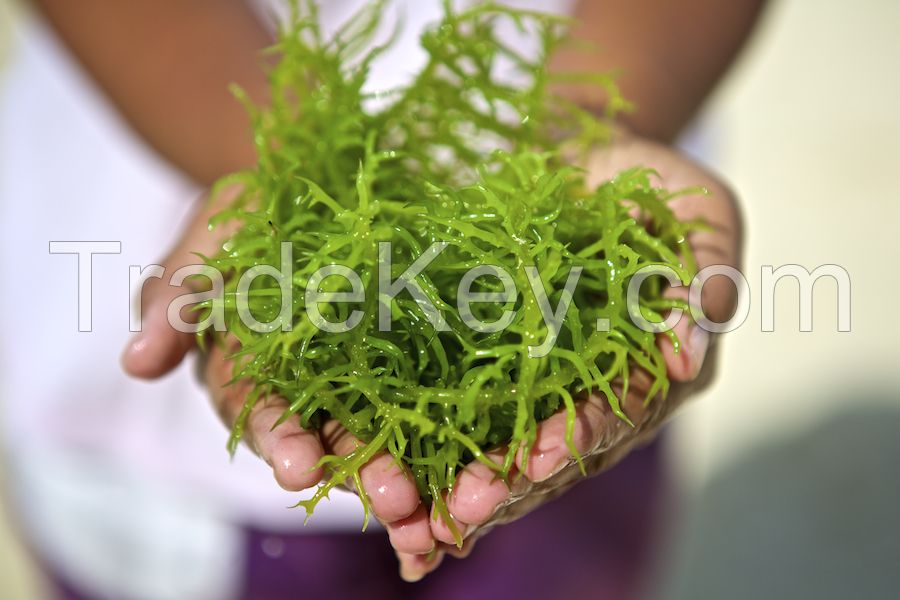The image is a rectangular photograph featuring a close-up of two wet, cupped hands holding a bright green, slimy plant substance that resembles seaweed or possibly dressed lettuce. The hands, which have a delicate, feminine appearance, are displayed prominently in the center of the frame. The person holding the plant is wearing a white shirt and purple pants. The background is blurred, revealing only a white wall with some shadows, contributing to the focus on the hands and the greenery. Overlaid in white text across the middle of the image is the watermark "TradeKey.com," suggesting the photograph could be an advertisement or stock image related to the website TradeKey.com. The colors in the image include shades of green, white, purple, brown, gray, and off-white.